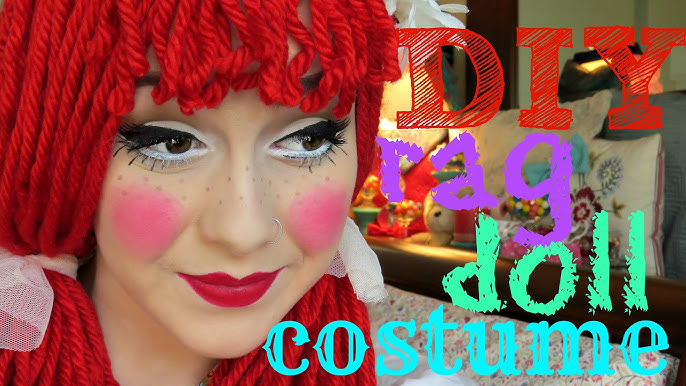This image, seemingly a thumbnail from a YouTube video, features a young girl intricately dressed as a ragdoll. She has striking reddish yarn hair, styled in two ponytails tied with white ribbons, reminiscent of Pollyanna or a vintage ragdoll. Her face is heavily made-up with thick eyeliner, mascara, white eyeliner beneath her eyes, and painted on freckles. She sports bright red lipstick and two distinct pink blush circles on her cheeks, highlighting her doll-like appearance. She has a nose ring complementing her heavily stylized makeup. To the right of the image, in a colorful font, reads "DIY ragdoll costume" with "rag" in purple, "doll" in green, and "costume" in turquoise. The background reveals an artfully designed room with a gumball machine, a table, a teddy bear, and an embroidered pillow, adding a cozy, playful atmosphere to the scene.